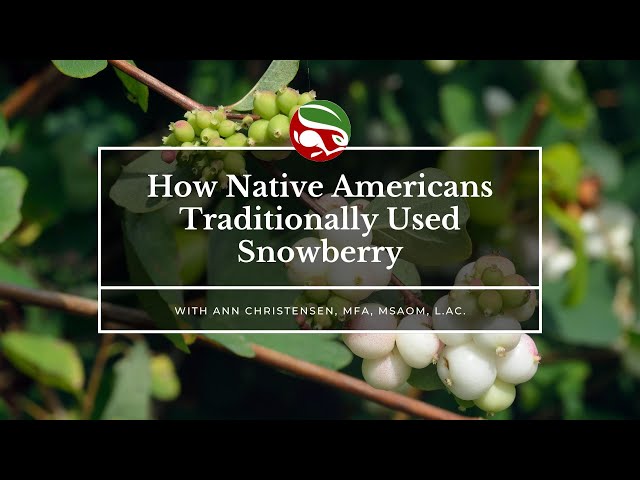The image appears to be the header of an article titled "How Native Americans Traditionally Used Snowberry," authored by Anne Christensen MFA, MSAOM, L.Ac. The title is displayed in white text within a transparent box outlined by a white border. Above the title, there is a small, stylized logo resembling a rabbit, which is white with a green section on top and a red section on the bottom.

The background features clusters of snowberries, with white and some green berries adorning a branch. Additional branches and leaves fill the background, creating a natural and dense backdrop. The image is framed by two black bars at the top and one at the bottom, giving it a bordered appearance.